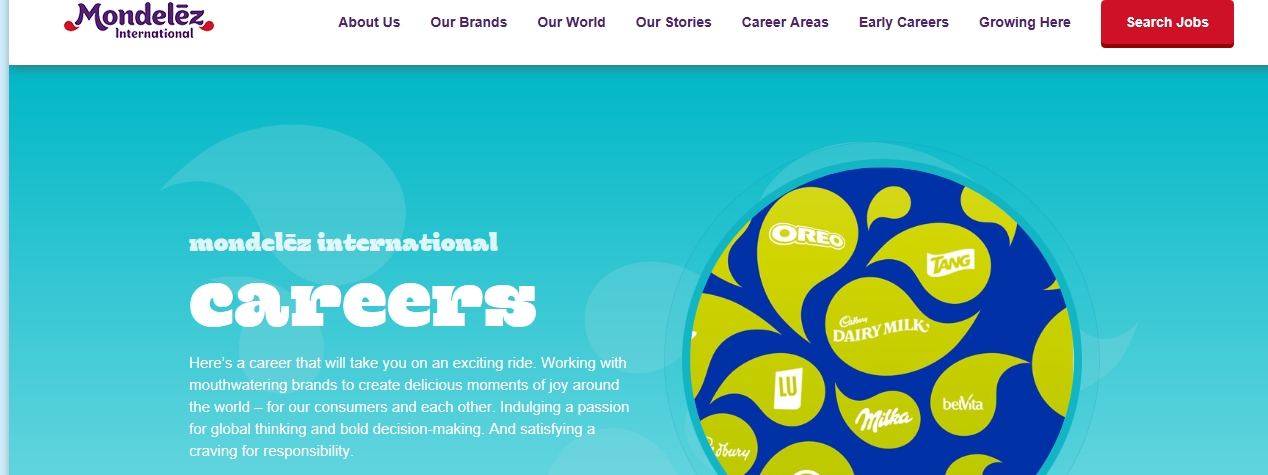Image Caption:  
The image is a screenshot from a website labeled "Mondelēz International," with the company name prominently displayed at the top in a white area. The name "Mondelēz" is spelled M-O-N-D-E-L-E-Z, with an accent over the final 'E.' The letters 'M' and 'Z' feature a distinctive design element, each adorned with red water droplet graphics.

Below the company name, there is a navigation menu with the following options: "About Us," "Our Brands," "Our World," "Our Stories," "Career Areas," "Early Careers," "Growing Here," and "Search Jobs." The "Search Jobs" option is highlighted within a red rectangle containing white text.

The lower section of the image has a teal background with a layered design resembling water droplets. On the left side, an orb encloses text in the shape of tear drops or water droplets, showcasing the brands Oreo, Dairy Milk, Tang, Milka, Belvita, among others. A detailed paragraph about career opportunities within Mondelēz International is positioned nearby, providing insight into the company's career offerings.